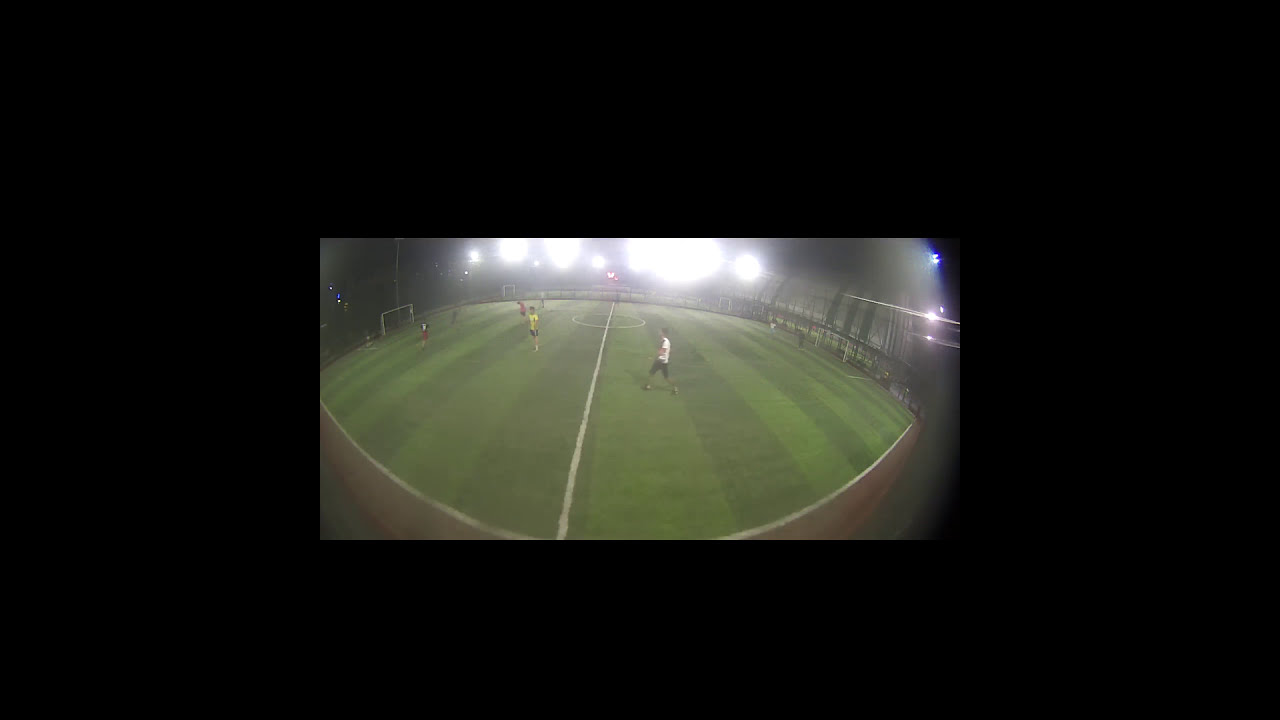This photograph captures a nighttime scene of a soccer field under bright stadium floodlights. The field, with its green grass and clearly marked white lines, is taken from mid-court, prominently featuring a white stripe stretching down the center and a circular mark denoting the halfway point. On each end of the field stand the soccer goals. 

Various players are scattered across the field, engaged in what seems to be a soccer game. One player, distinctively dressed in a white short-sleeve shirt and black shorts, along with black and white tennis shoes, stands out. Another player, in a yellow short-sleeve shirt and black shorts, is also visible among the group. There’s a notable presence of players in red attire, particularly concentrated on the left side of the center line.

The floodlights tower above, casting powerful illumination on the entire scene and creating a stark contrast against the dark, night sky. The surrounding bleachers, although not heavily detailed, frame the grassy expanse and provide context to the stadium setting, with a few lights emitting a bright blue hue, adding an extra dimension to the nighttime ambiance. The photograph appears slightly concave, perhaps due to the lens, giving the field a rounded appearance despite its true flatness. All these elements together craft a vivid, detailed depiction of a nighttime soccer game in progress.